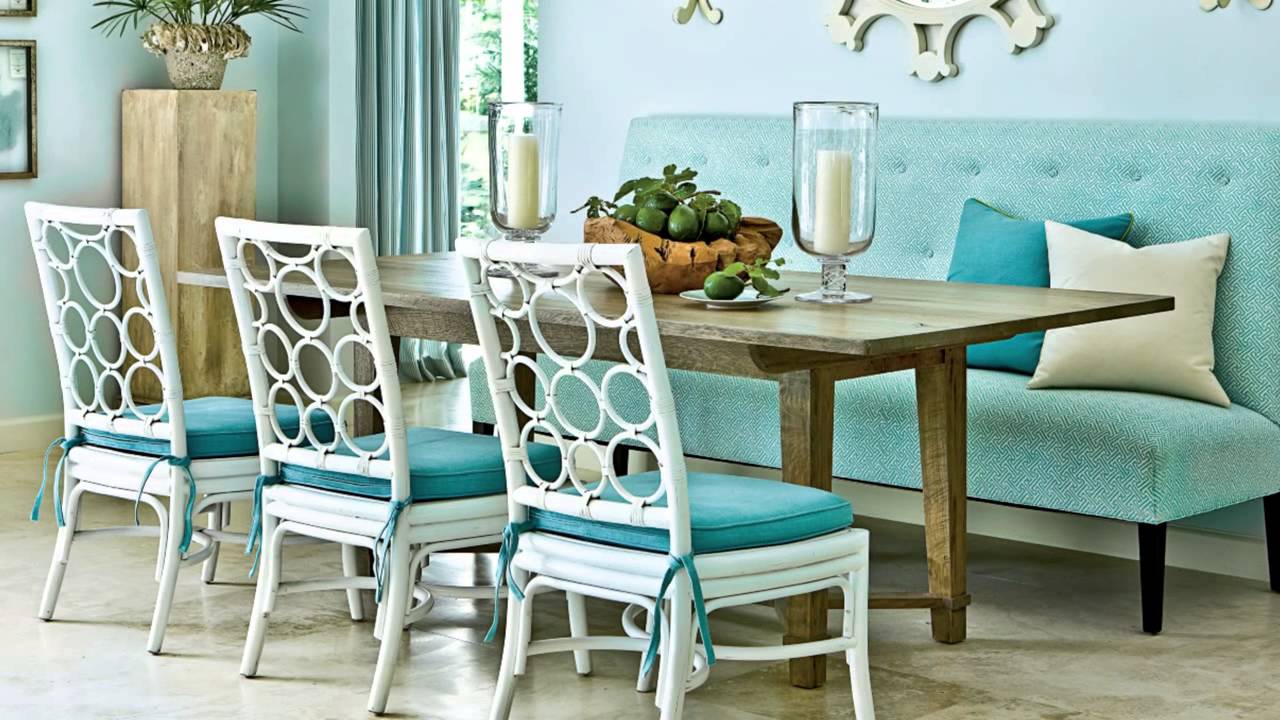This photograph captures a modernistic indoor dining room bathed in natural light. The walls are painted a serene, sky blue, complementing the minimalist aesthetic of the room. Against the far wall, there is a light teal bench with a high back, adorned with two throw pillows—one cream and one dark teal. In front of the bench stands a sleek, minimalist wooden dining table. At the center of the table, a fruit basket filled with limes is flanked by two 3-inch pillar candles housed in glass vases.

On the opposite side of the table, there are three white chairs featuring a circular pattern on the back, each cushioned with teal fabric. The floor beneath is a chic gray concrete, adding to the contemporary feel of the space. To the left of the table, a four-foot-tall column supports a faux palm plant, enhancing the room's tranquil atmosphere. Additionally, a sliding glass door in the corner and a couple of pictures on the wall complete the setting, adding to the airy, welcoming ambiance of this stylish dining area.